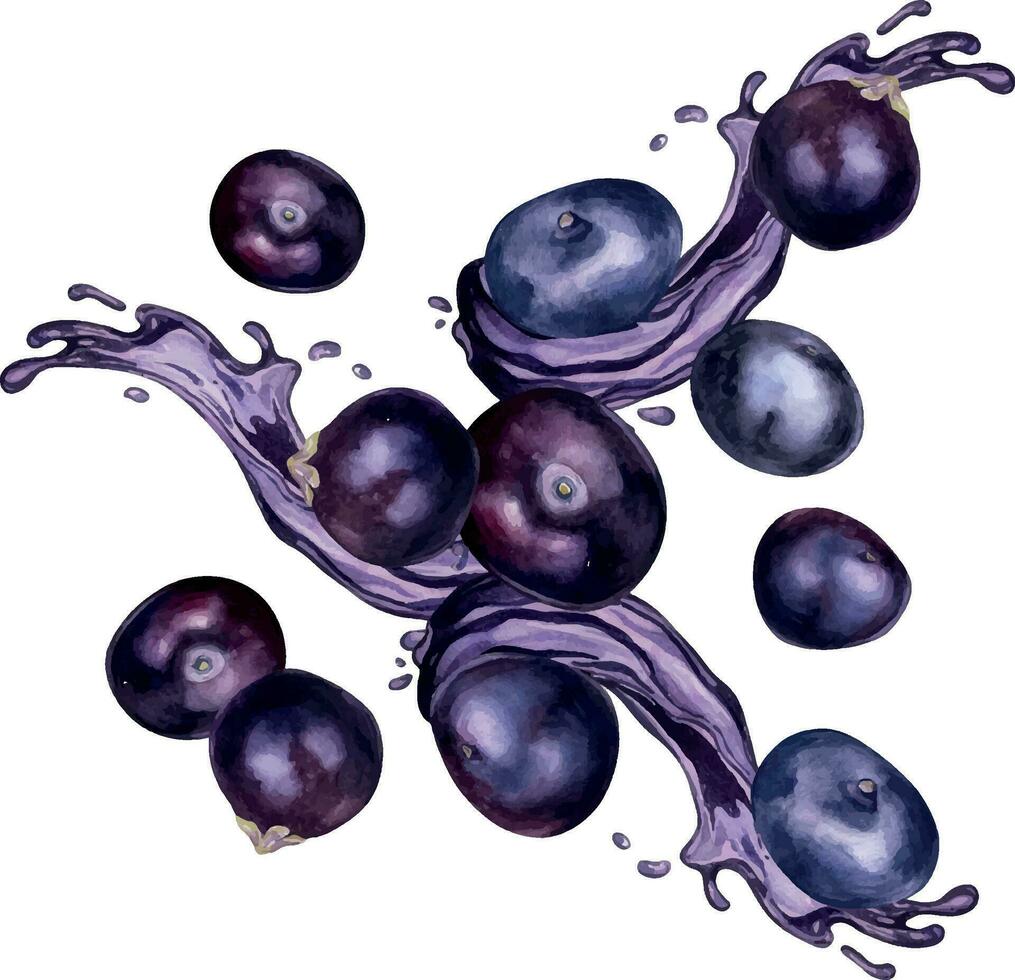This illustration features a hand-drawn depiction of approximately 13 blueberries, rendered in a watercolor style with splotchy, watery colors on a clean white background. The blueberries, varying in shades of rich purple and blue, appear glossy with hints of light reflecting off their surfaces. Scattered in different orientations and sizes, some blueberries are adorned with green leaves, adding to their organic appearance. A purple, translucent liquid encircles several central berries, creating a dynamic splash that wraps around them like a swirling tornado. This liquid extends diagonally across the image, adding movement and emphasizing the fruit's juicy nature.